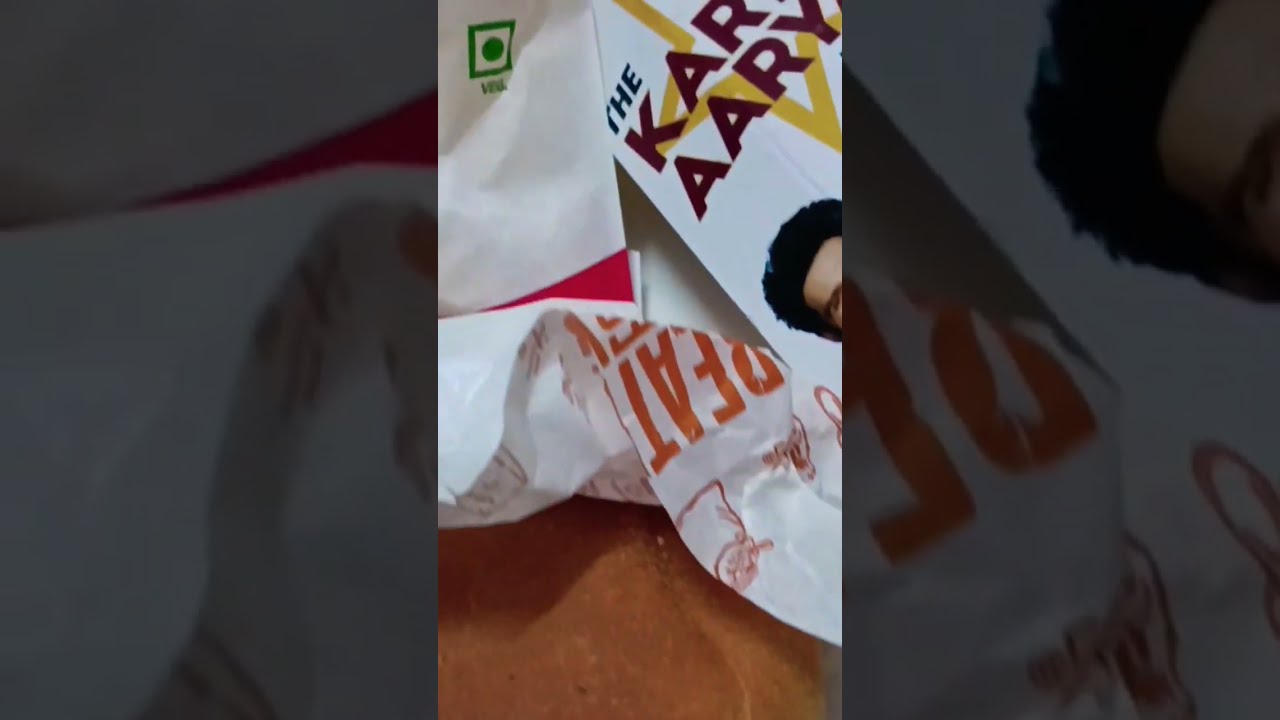This image shows a close-up view of several crumpled wrappers and containers, arranged haphazardly on a brown wooden surface. The centerpiece is a wrinkled white paper or wrapper featuring a mix of colored sections in green, yellow, maroon, and orange. A notable detail is the partially visible, large orange word "beat" on one of the wrappers. Above it, partially cut off by the image's frame, are other containers that remain mostly out of view. The setting appears to be indoors, potentially on a counter or kitchen table, under soft lighting. The overall composition gives a cluttered and informal impression, as if the items were discarded carelessly. The image has a horizontal rectangular orientation, with dark gray shading on both vertical sides, suggesting it could be a screenshot from social media like TikTok or Instagram. Additionally, there are faint, unreadable texts on some wrappers, one of which seems to depict part of a man's face. The scene seems to convey an everyday, perhaps slightly messy, moment captured through a digital lens.